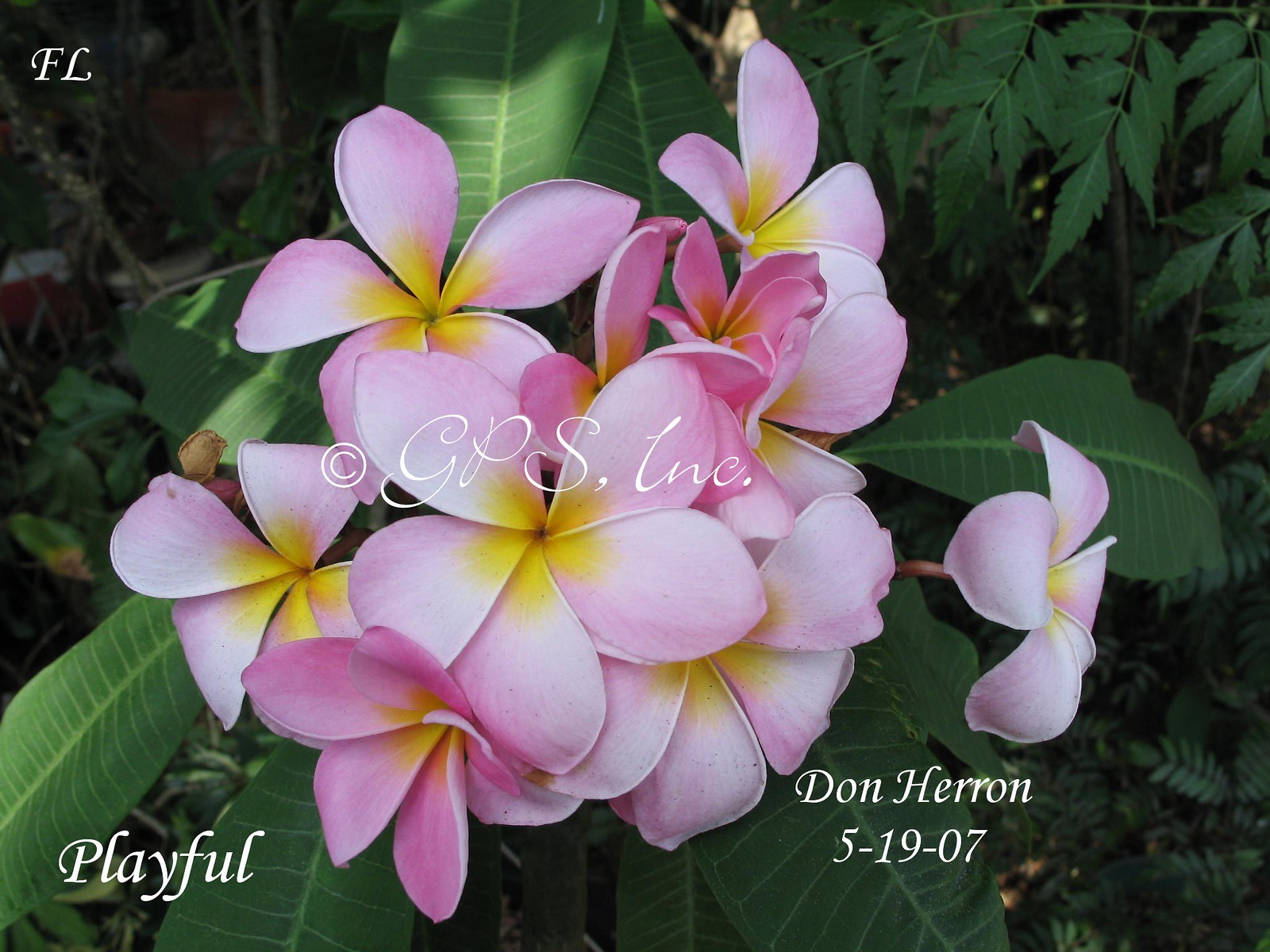The image is a close-up shot of a central pink flower with shades ranging from light to dark pink, accented by bright yellow centers. The flower dominates the center of the image, surrounded by thick, dark green leaves. In the background, various smaller bushes, leaves, and possibly trees suggest an outdoor garden setting, likely photographed in the middle of the day. Text details include "F.L." in the upper left corner, "playful" in white letters in the lower left corner, and "Don Heron 5-19-07 at JPS Inc." in the lower right corner beneath the petals. The overall scene is vibrant with colors including pink, purple, yellow, green, black, and white.